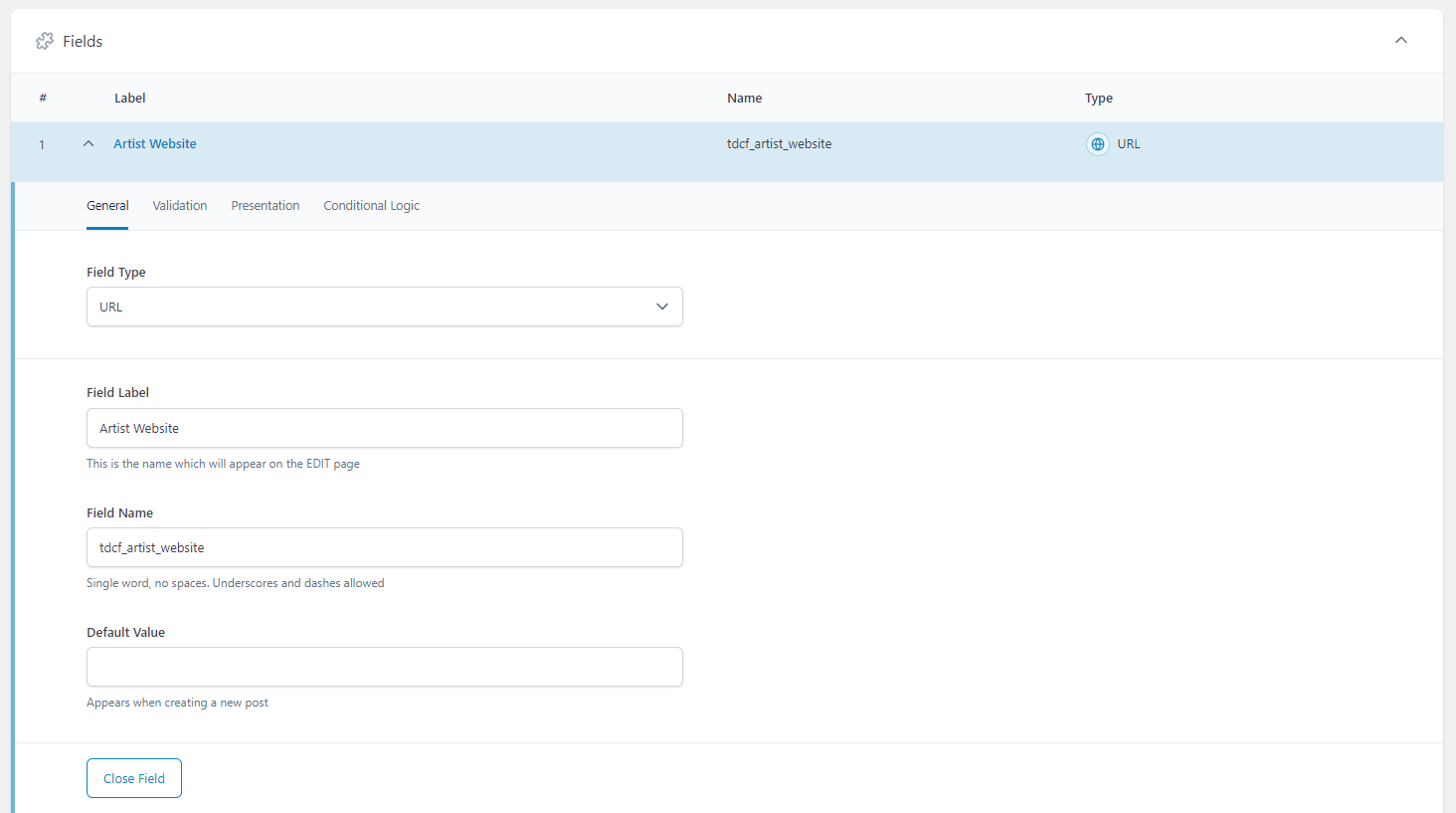This image is a screenshot of a low-quality website interface, making the text somewhat challenging to read. The interface is bordered on the left, right, and top by a narrow gray bar. At the very top, there is a white vertical rectangle. In the top-left corner, there is black text labeled "Fields," accompanied by a small, indiscernible icon. The top-right corner features a small black arrow pointing upward.

Beneath the top section, there is a gray rectangle with black text displaying "Label," "Name," and "Type." Directly below this, a blue rectangle presents corresponding values: under "Label" is "Artist Website," under "Name" is "Todd Artist Website," and under "Type" is "URL."

Further down, another gray rectangle features the word "General," which is selected and underlined in blue. Next to it are options labeled "Validation," "Presentation," and "Conditional Logic." The "General" tab is open, revealing a white-background section titled "Field Type," with a drop-down menu showing "URL." Below this, another section labeled "Field Label" contains a drop-down menu displaying "Artist Website" and an explanatory note stating, "This is the name which will appear on the edit page." Lastly, the "Field Name" section shows the text "T Todd Artist Website."